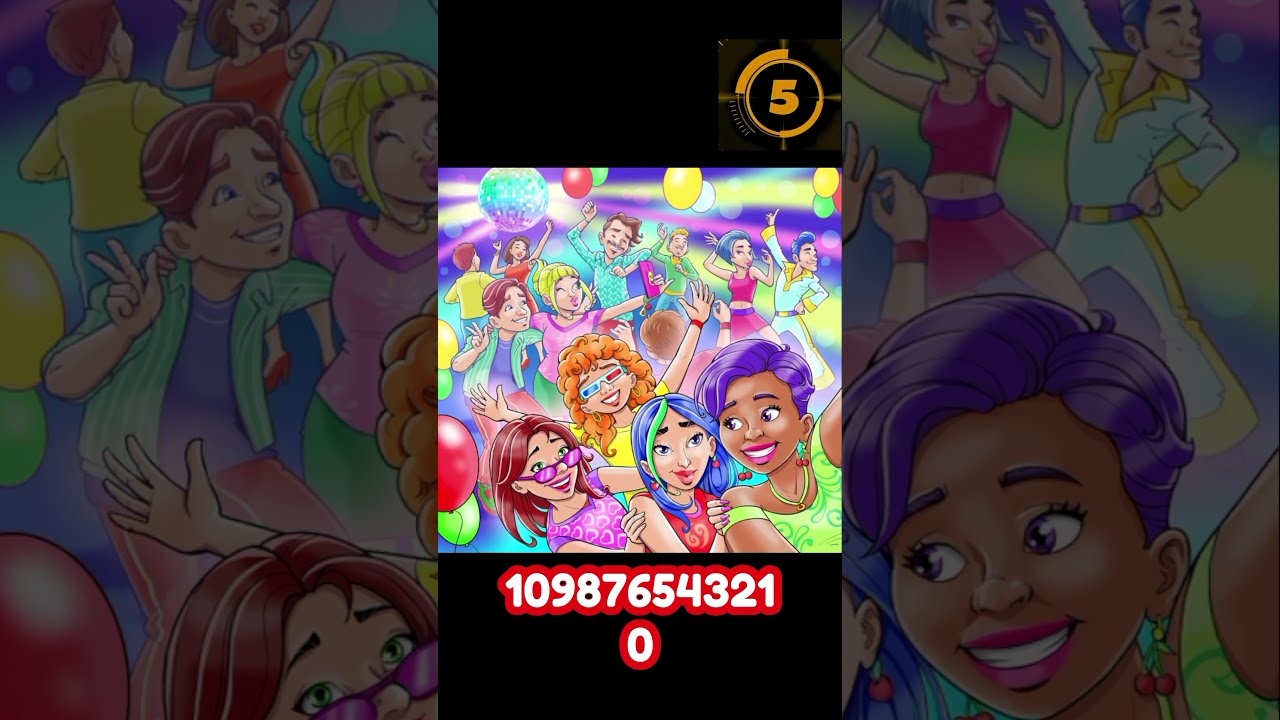In this vibrant, cartoon-style image, a lively New Year's Eve dance party unfolds with a dynamic array of colorful characters and decorations. Dominating the foreground is a diverse group of women: a girl wearing a purple dress and matching shades with brown hair, a girl in a red shirt with striking blue and green hair, another in a green dress with short purple hair, and a girl in a yellow dress with curly orange hair donning 3D glasses. 

Above them, a disco ball in the upper left corner sends out shimmering red, orange, and yellow rays, illuminating the scene. Balloons float through the air, adding to the festive atmosphere. In the background, several individuals, including a man in an Elvis suit, join the dance, contributing to the energetic vibe.

The image is set against a dominating red background, featuring a white numeral countdown from 10 to 0 at the bottom, where the final "0" is placed on a second row by itself. In the upper right corner, a prominent gold circle with the number 5 inside serves as a dial-like graphic element. 

On both sides of this portrait-oriented illustration, the main image is repeated in close-ups with a black opaque overlay, showcasing the exuberant partygoers in more detail. This carefully crafted cartoon scene captures the joyous and spirited essence of a New Year's Eve celebration.